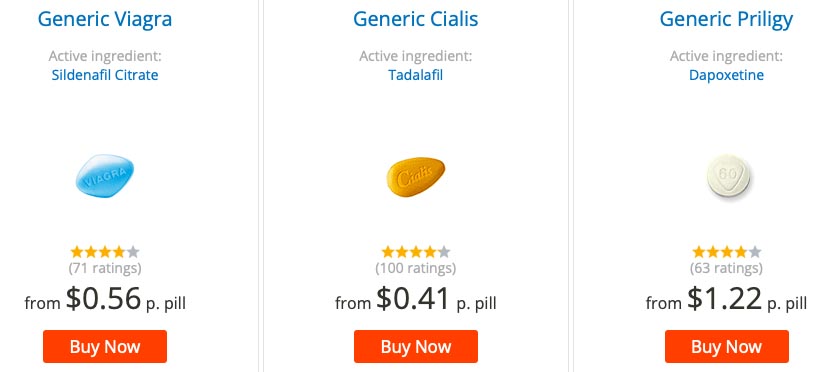The image features a white background with three different medications showcased, as found on a pharmacy website. 

- On the left side:
  - In blue text: "Generic Viagra"
  - In gray text: "Active Ingredient"
  - In blue text: "Sildenafil Citrate"
  - Below this information, a blue, diamond-shaped tablet is displayed.
  - The medication has a rating of 4 out of 5 stars from 71 ratings.
  - Pricing is listed as starting from 56 cents per pill.
  - There is a red button with white text saying "Buy Now".
  
- In the center:
  - In blue text: "Generic Cialis"
  - In gray text: "Active Ingredient"
  - In blue text: "Tadalafil"
  - Below this information, a small, brown, triangular-shaped pill is shown.
  - The medication has a rating of 4 out of 5 stars from 100 ratings.
  - Pricing starts from 41 cents per pill.
  - It also features a red "Buy Now" button.

- On the right side:
  - In blue text: "Generic Prilogy"
  - In gray text: "Active Ingredient"
  - In blue text: "Depoxetine"
  - Below this information, a small, round, white pill is depicted.
  
Each medication section provides essential details, including the active ingredient, user ratings, price per pill, and a purchasing option via a prominent red "Buy Now" button.